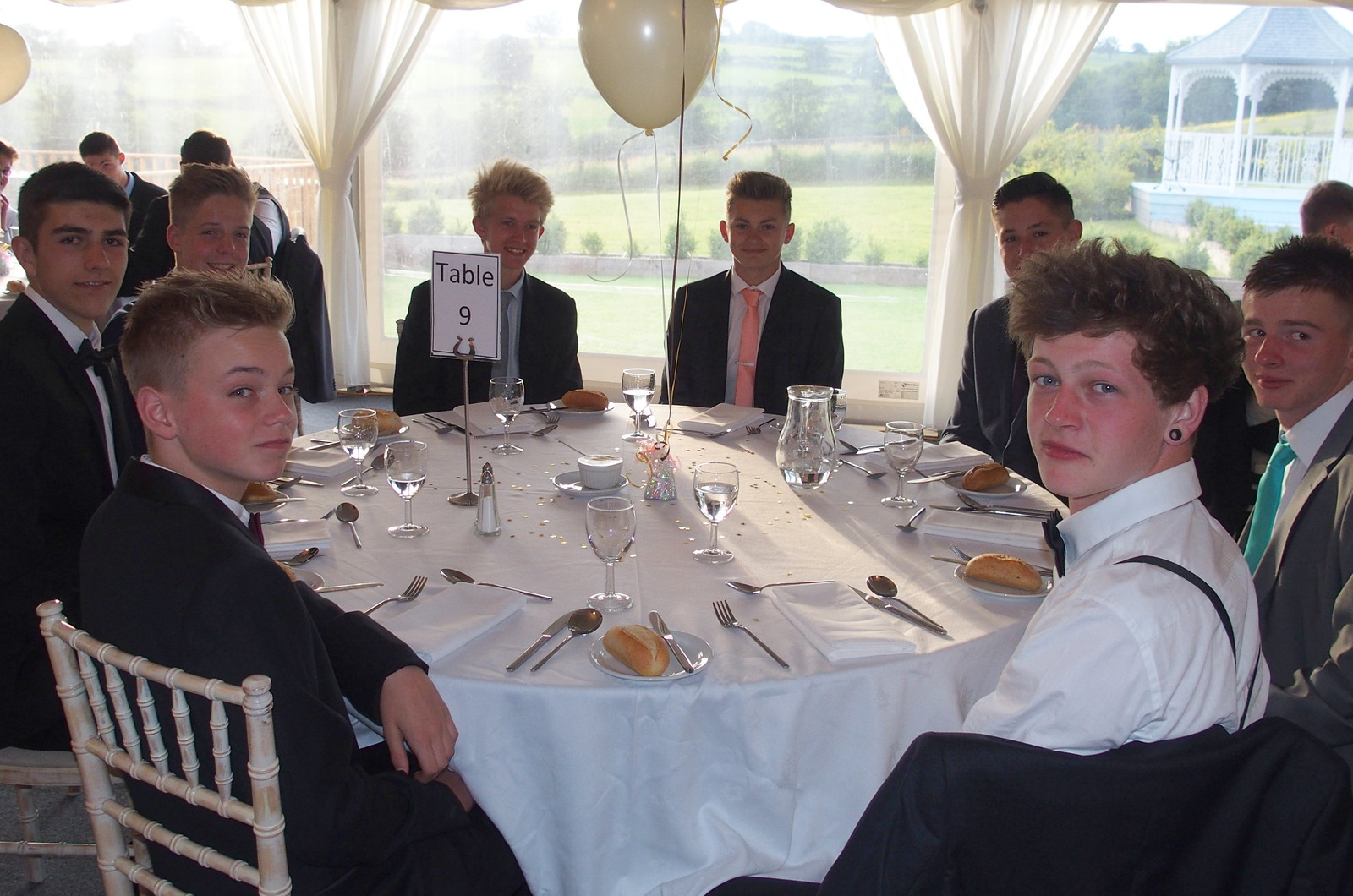This color photograph captures a formal outdoor event with a round table of eight young men, who appear to be high school age, dressed in dark suits with white shirts, sitting under a canopy. They are gathered around Table 9, as indicated by a white place card. Each person at the table has a distinct look: one wears a pink tie, another a blue tie, and another a green tie, while one young man has his suit jacket draped over his chair and is dressed in black suspenders, a white shirt, and a black bow tie. A few of them have short hair in various shades—blonde, dark brown, and reddish. One young man has pierced ears. On the white tablecloth-covered table, there are clear water glasses, a pitcher of water, napkins, silver cutlery, and each place setting includes a small bun on a saucer. In addition to these items, a salt shaker is also visible. Cream-colored helium balloons float above the table, adding to the festive atmosphere. In the background, a gazebo can be seen in the top right corner of the image, enhancing the outdoor venue's charm. The young men are looking towards the camera, adding a lively and engaging element to the photograph.